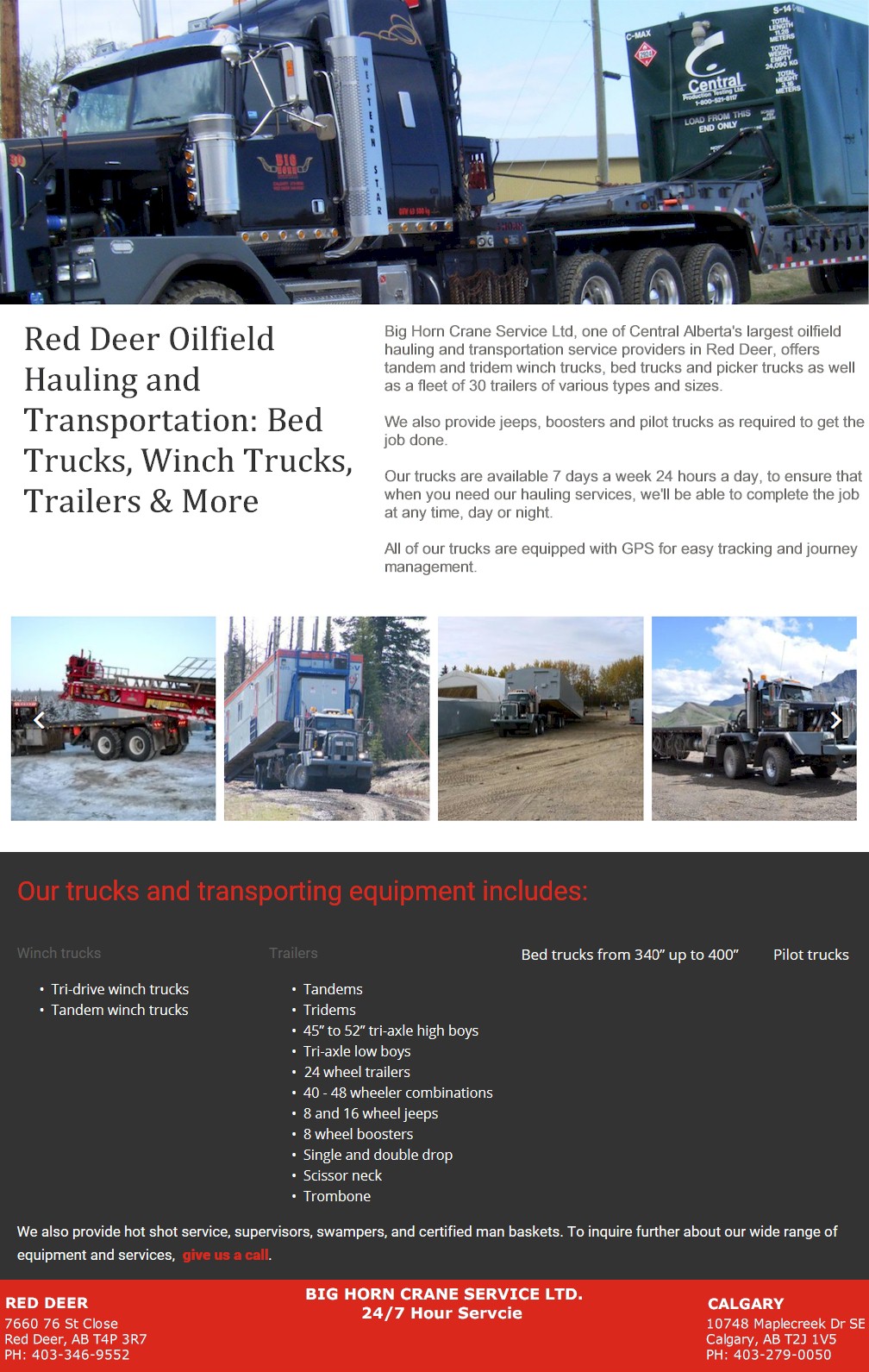This image showcases a sleek, black semi-truck featured on a website dedicated to semi-trucks and transportation services. The truck is part of the fleet belonging to Big Horn Crane Service, LTD, a leading oil field hauling and transportation service provider based in Red Deer, Central Alberta. The company boasts a wide range of vehicles and equipment, including tandem and tridem width trucks, bed trucks, picker trucks, and a diverse fleet of 30 different trailers.

Big Horn Crane Service, LTD, offers 24/7 service and provides additional support such as hot shot services, field supervisors, swampers, and certified man baskets. For more information or inquiries about their extensive equipment and services, you can visit them at 7660 76 St. Close, Red Deer, AB T4P 3R7, or call them at 403-346-9552.